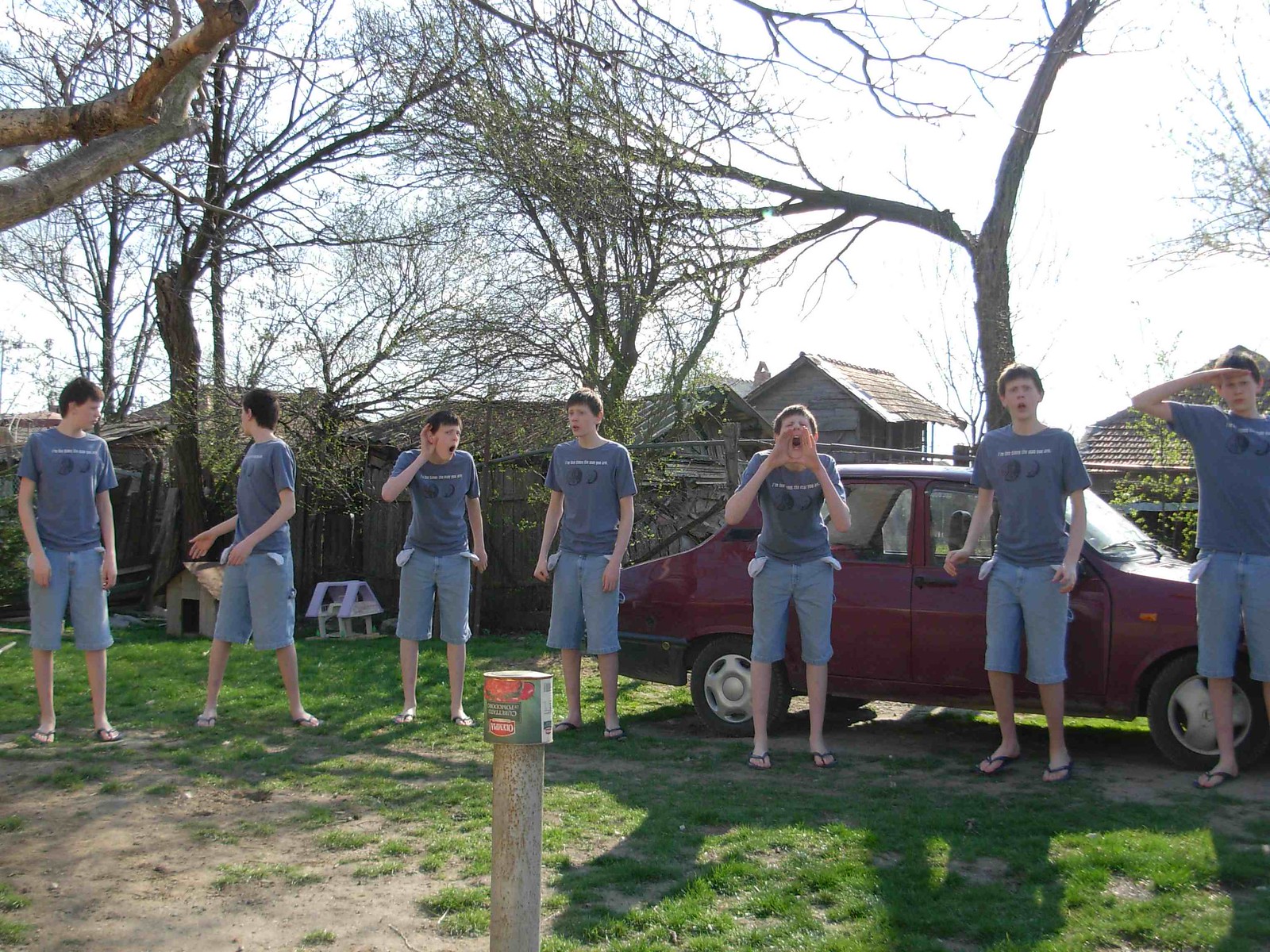This color photograph, taken in landscape format, captures a backyard scene during daytime. The backdrop includes a patchy lawn with a mix of grass and dirt, a maroon car parked off to the right on the lawn, and a wooden privacy fence with trees and other houses visible in the distance. A notable feature in the yard is a small wooden doghouse near the fence. The main focus of the image is an intriguing visual effect: seven identical adolescent boys, each with dark brown hair and a fair complexion, are seen standing in various poses across the yard. 

Each boy is dressed identically in gray cargo shorts with pockets turned out to reveal the white linings, black thong sandals, and light gray t-shirts with an indistinguishable black image and white text. Despite their identical appearances, each boy adopts a unique pose—one shielding his eyes from the sun, another cupping his mouth as if shouting, and a third with his hand to his ear, among others looking in different directions. These boys are, in fact, the same individual captured in multiple instances and merged into one image using special effects, creating a captivating portrayal of the same boy in different poses and positions within the same yard.